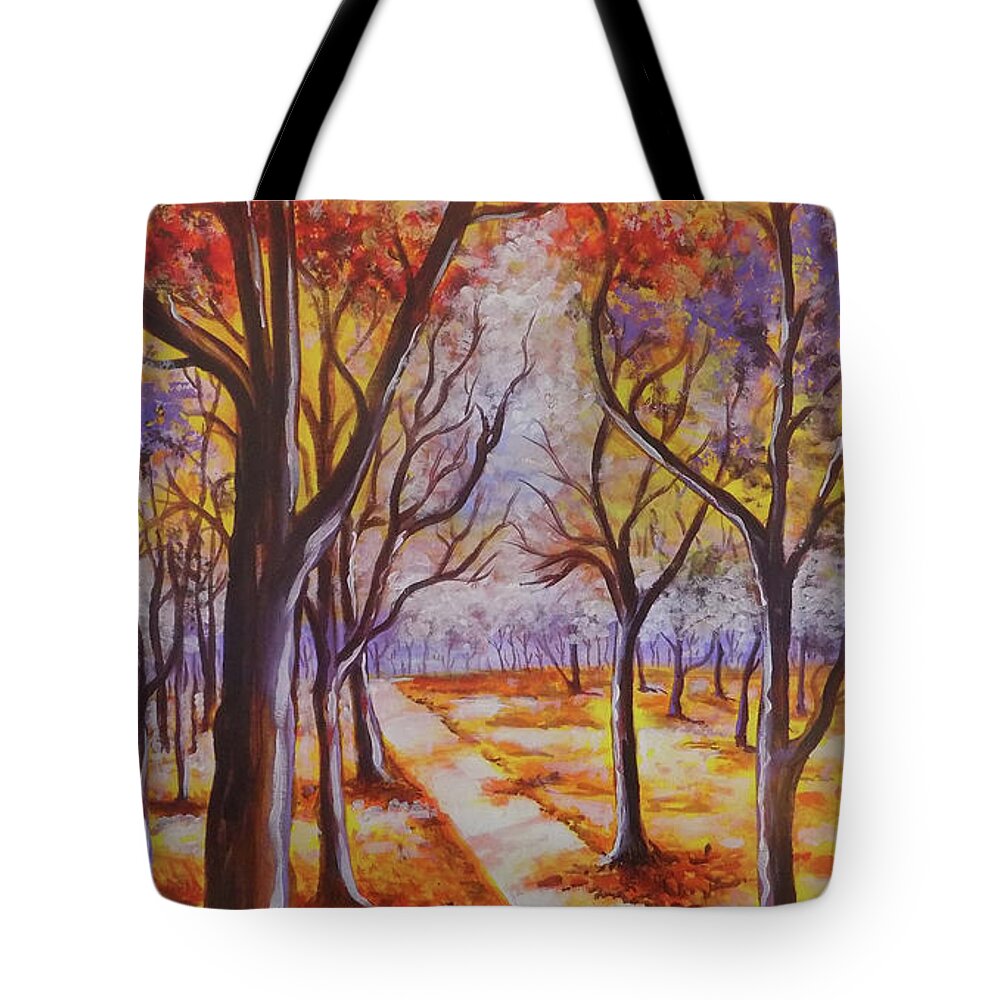This image showcases a top-down view of a tote bag set against a white backdrop. The tote bag features a unique and detailed painted scene of a fall forest. The design predominantly displays various trees with darker, almost blackish-brown trunks, and vibrant foliage in hues of yellows, golds, reds, and occasional purples, suggesting the autumn season. The tree leaves exhibit a blend of colors, including yellowish tones predominantly in the foreground, transitioning to reddish hues, and whites as the scene approaches the horizon. The ground underneath the trees appears golden and yellow, possibly covered in fallen leaves, contrasting with a concrete path meandering through the center. Smaller trees with thinner stumps and white leaves can be seen towards the back, against a subtly faded blue sky. The bag’s black strap is partially visible. The entire scene is animated and artistic, employing a colorful and somewhat abstract palette, giving it a distinct fall-like ambience. This image likely represents an advertising demonstration of a company’s ability to print detailed and vibrant scenes onto tote bags.